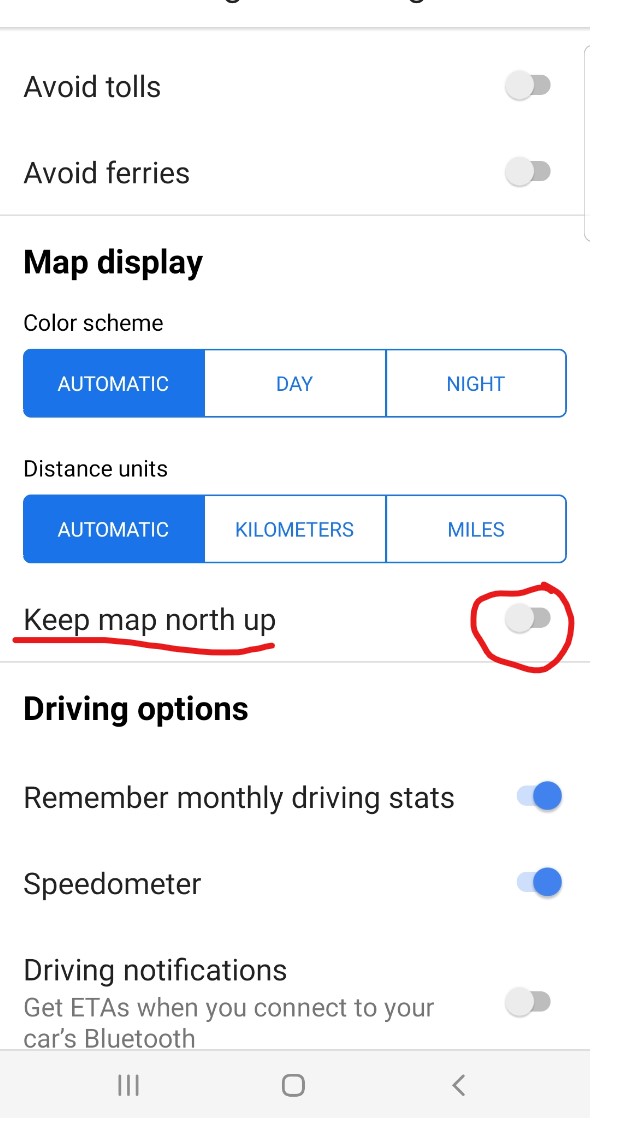This image is a slightly cropped screenshot taken from a mobile device, specifically from the navigation settings in the map application. The bottom of the screenshot features a light grey bar containing three icons resembling those on Apple mobile devices: three vertical lines, a square, and a backward arrow.

The main content of the screenshot displays a list of options for the navigation route. At the top, there are two toggle sliders labeled "Avoid tolls" and "Avoid ferries". Below these sliders, there are options to select a color scheme for the map display: Automatic, Day, or Night. Additionally, users can choose the distance units from options such as Automatic, Kilometres, and Miles.

Another slider option, labeled "Keep map up north," is currently turned off. This specific slider has been highlighted with a red underline and encircled with a red circle for emphasis.

Further down, the driving options section shows three toggles. The first two options, "Remember monthly driving stats" and "Speedometer," are switched on, while the third option, "Driving notifications," is turned off.